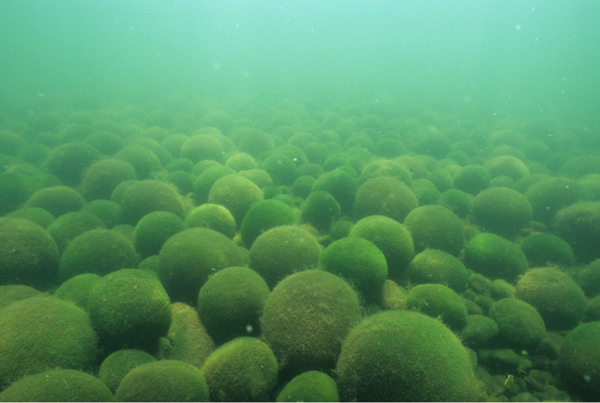The image depicts an underwater scene with a murky, green aquatic environment, suggesting a lake bed. The water is a gradient of greens and blues, turning almost aqua at the top, indicating the presence of sunlight filtering through the shallow depths. The lake floor is densely packed with variously-sized spherical objects that appear to be rocks or stones enveloped in vibrant green and yellow moss or algae. These objects create a texture reminiscent of fuzzy green balls or hairy coconuts, carpeting the entire expanse from left to right and stretching out to the horizon, beyond which the view becomes indistinct due to the haziness of the water. The lack of air bubbles or other aquatic life provides an eerie, surreal quality to the scene.